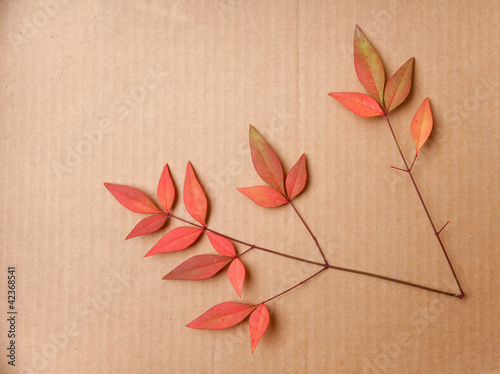This image features a brown cardboard background entirely filled with "Adobe Stock" watermarks, which are diagonally oriented from bottom left to top right, and a specific watermark with the number 42368541 written sideways in the bottom left. Dominating the bottom right are two thin branches with reddish-orange autumn leaves, some tinged with green. The branches diverge at the bottom right, one extending diagonally at approximately 85 degrees and the other at about 50 degrees to the left. The leaves are clustered primarily in groups of three at the ends of various branchlets, though a couple of branchlets are leafless, and one has a solitary leaf. The branches themselves are reddish in color.